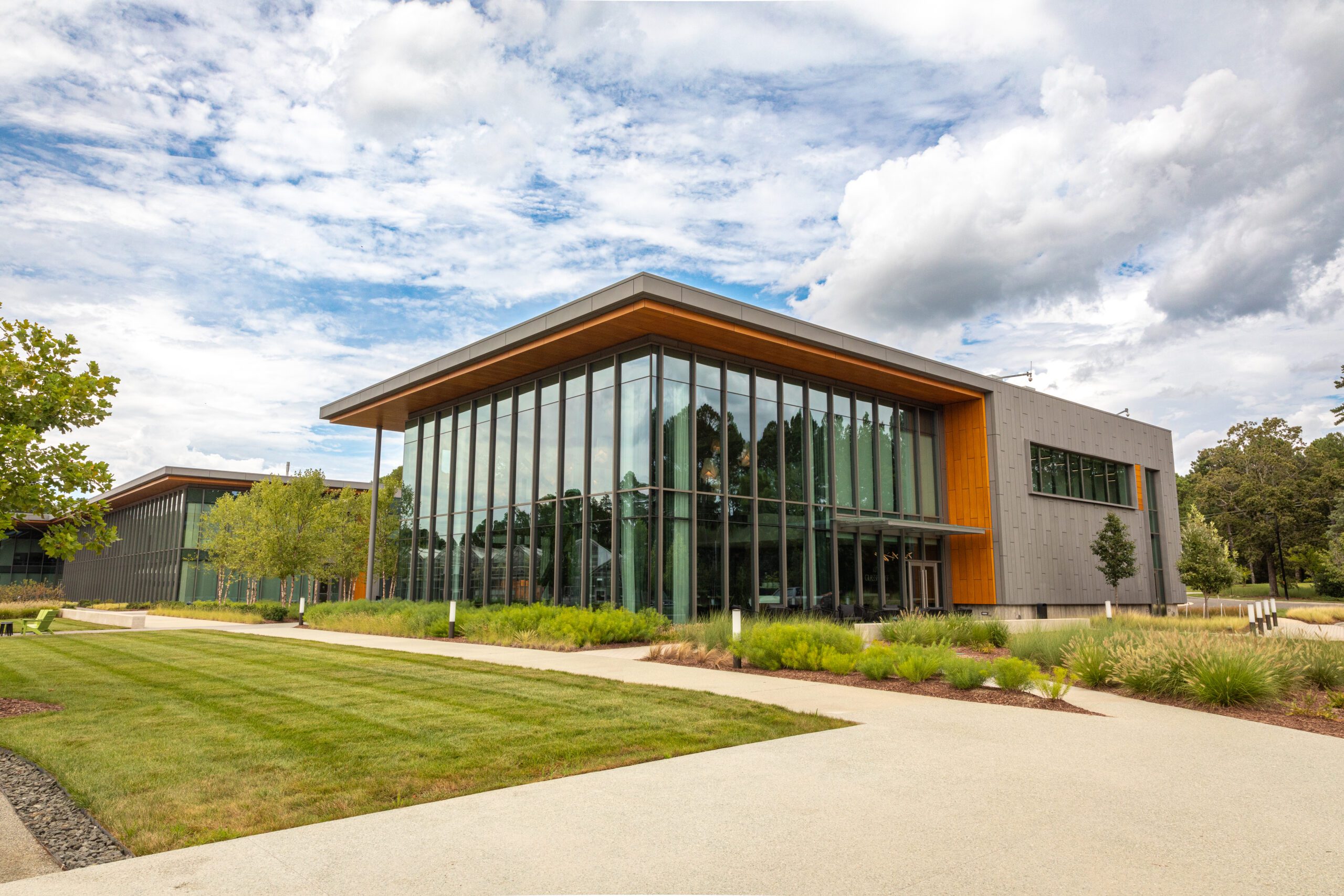This image features a contemporary building, potentially an office, library, school, or science museum, captured from the lawn in front of the entrance. The front section prominently displays floor-to-ceiling glass windows on three sides, accentuating its modern aesthetic. The other half of the building showcases sleek gray paneling with windows located higher up. Notably, the structure is supported by numerous slender, brownish steel columns and has an eye-catching orange soffit. In front of the building stretches a spacious concrete expanse and a well-maintained grass lawn, dotted with freshly planted green shrubs and benches. Adjacent to this building is an identical structure, reinforcing the campus-like setting. The scene includes a driveway, glimpses of parked cars, and a partially visible tree, with the background featuring many trees and a cloudy sky. This detailed arrangement of elements conjures images of a vibrant, functional college campus or possibly a group of modern office buildings.